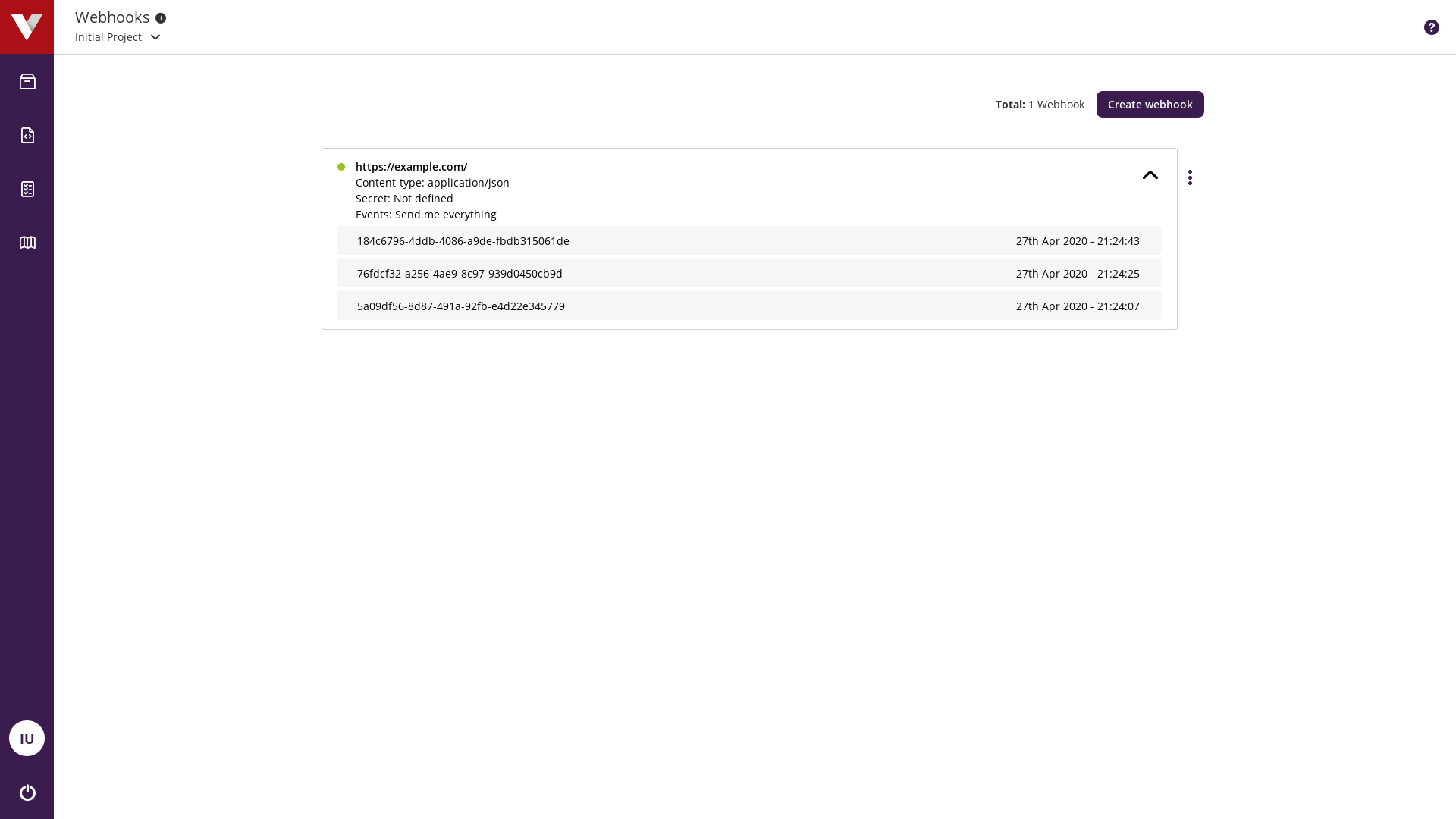The image displays the Webhooks website interface. At the top of the page is a white banner featuring the word "Webhooks" accompanied by a black dot. Below this banner, there is a section labeled "Initial Project" with a small font size, making it slightly difficult to read. This section includes a drop-down arrow. Towards the right side of the banner, there is a black circle containing a white question mark, indicating a help or information icon. 

On the far left, a vertical blue border runs down the page. At the top of this border, there's a red square icon with a two-tone 'V' inside it. Below this, a series of icons line the border, including a shopping cart, a piece of paper, and a book, among others. Near the bottom of this vertical section, there's a profile icon with the initials "IU." Adjacent to this, an on-off switch icon is visible.

In the middle section of the webpage, the text "Total" is displayed, followed by "Webhook." To the right of this text is a rectangular "Create Webhook" button, which is blue in color. 

Below this section, there is a box starting with a green dot followed by an HTTPS address. This box contains three sections, each highlighted in light gray, likely indicating parts of the webhook configuration or information.